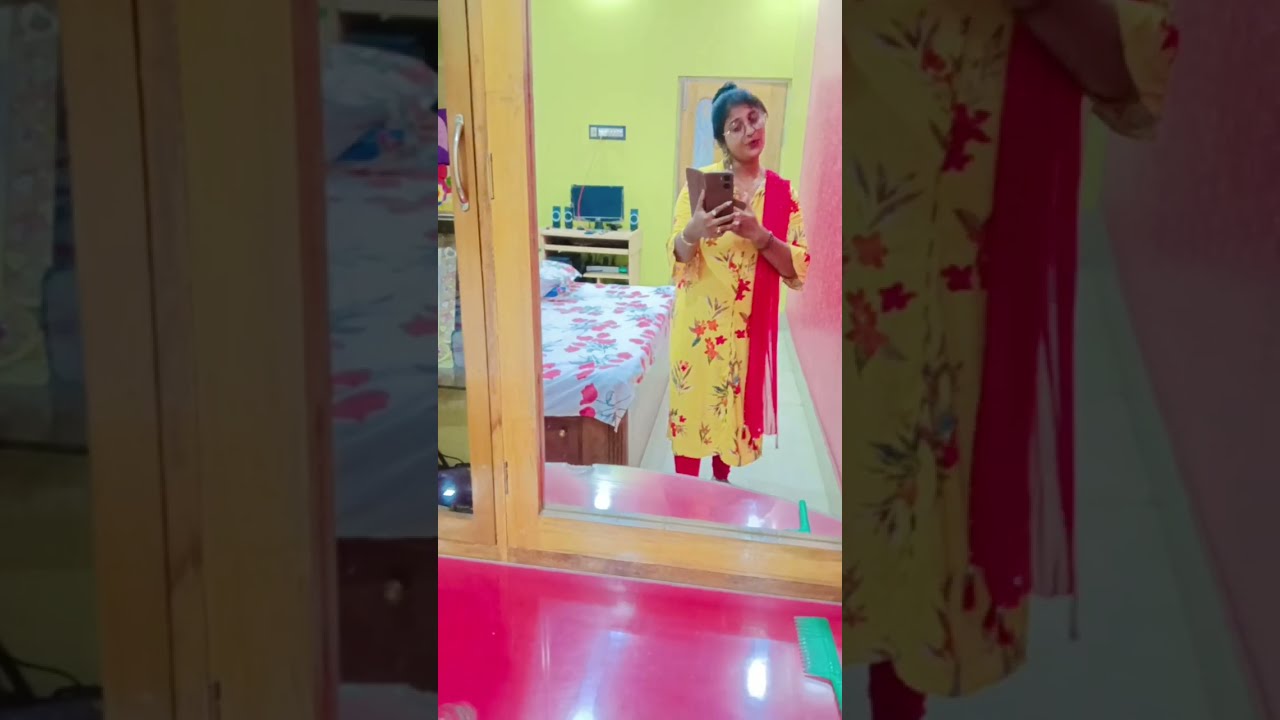The image features a middle-aged Indian woman with her hair styled in a bun and wearing glasses. She is standing in front of a mirror, holding a smartphone to take a selfie. She is dressed in a yellow sari adorned with red flowers and complemented by a long red scarf draped over her shoulder. A bracelet adorns her wrist. The setting is a tidy and clean bedroom with vibrant yellow walls and a mix of red alongside a wooden door. She stands next to a bed that has a white comforter with a red flower pattern. In the background, there is a computer with speakers on a desk or table console, suggesting she may have been engaged in some daily activity before deciding to capture the moment.